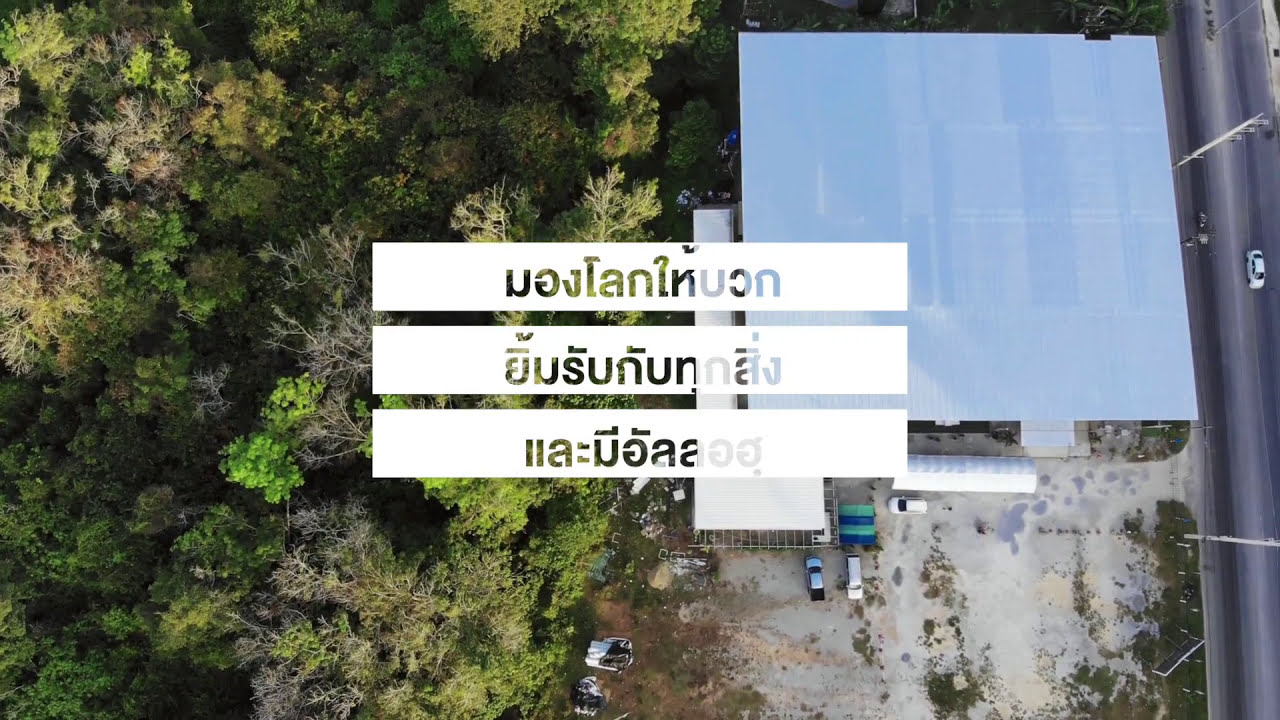This aerial photograph captures an expansive view from high above, showcasing a landscape dominated by lush, deciduous trees full of green leaves. At the center of the image, three rectangular boxes aligned vertically contain text in a foreign language, featuring unfamiliar characters resembling a backwards "U," an "A," an "N," and others. On the right side of the image, a large building with a distinct blue, possibly metallic, roof is visible. This building extends from the road on the right-hand edge of the frame, where a white car can be seen traveling on a paved, blacktop highway. Below this building, a dirt-covered and worn-out parking area is dotted with cars including a white bus and vehicles in white and light blue. Adjacent to this area are patches of green interspersed in the dirt, reflecting a less manicured terrain. To the left of the building and the parking lot, a dense collection of trees forms a vivid green canopy, enhancing the natural beauty of the scenery.